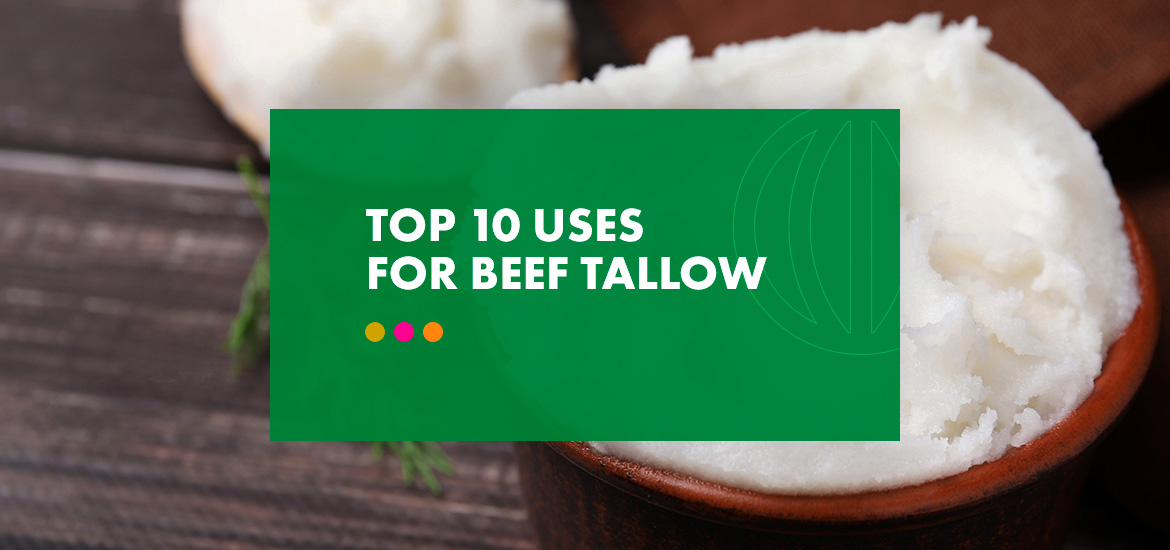The image is a detailed informational banner prominently featuring a green rectangular box in the center with white text that reads "Top Ten Uses for Beef Tallow." To the left of the text, there is a circular symbol with crescent-like cuts. Below the text, there are three dots: the first is a yellow-orange, the second is pink, and the third is a true orange. 

Behind the green banner is a visually engaging background that includes a bowl, likely made of wood or stone, filled with white, ground-up beef tallow. This bowl rests on a wooden table, and additional out-of-focus tallow can be seen in the background. The detailed and rich textures of the green box, text, and dots, combined with the natural elements of wood and tallow, create a visually appealing layout aimed at conveying information effectively.